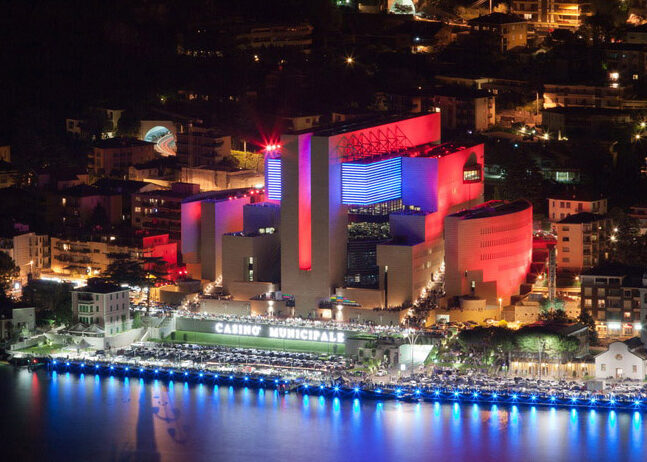An aerial nighttime photograph captures a brightly and colorfully lit building that prominently displays the sign "Casino Municipale" at its base. The casino's architecture is highly geometric, with various sections differing in size and shape, including rounded ends and stair-like features. The building's facade glows with hues of blue and red lighting, accented by some green lights below the sign. The central section of the casino, shaped like a 'U,' stands out amid the modern design. In front of the casino is a platform that appears to serve as a parking lot full of cars, positioned right at the water's edge. This platform is lined with bright blue lights that create a striking reflection on the water. The photo, likely taken by a drone, shows a backdrop of numerous smaller buildings ascending a hillside, indicating the casino is set in a nocturnal urban landscape, possibly in Italy.